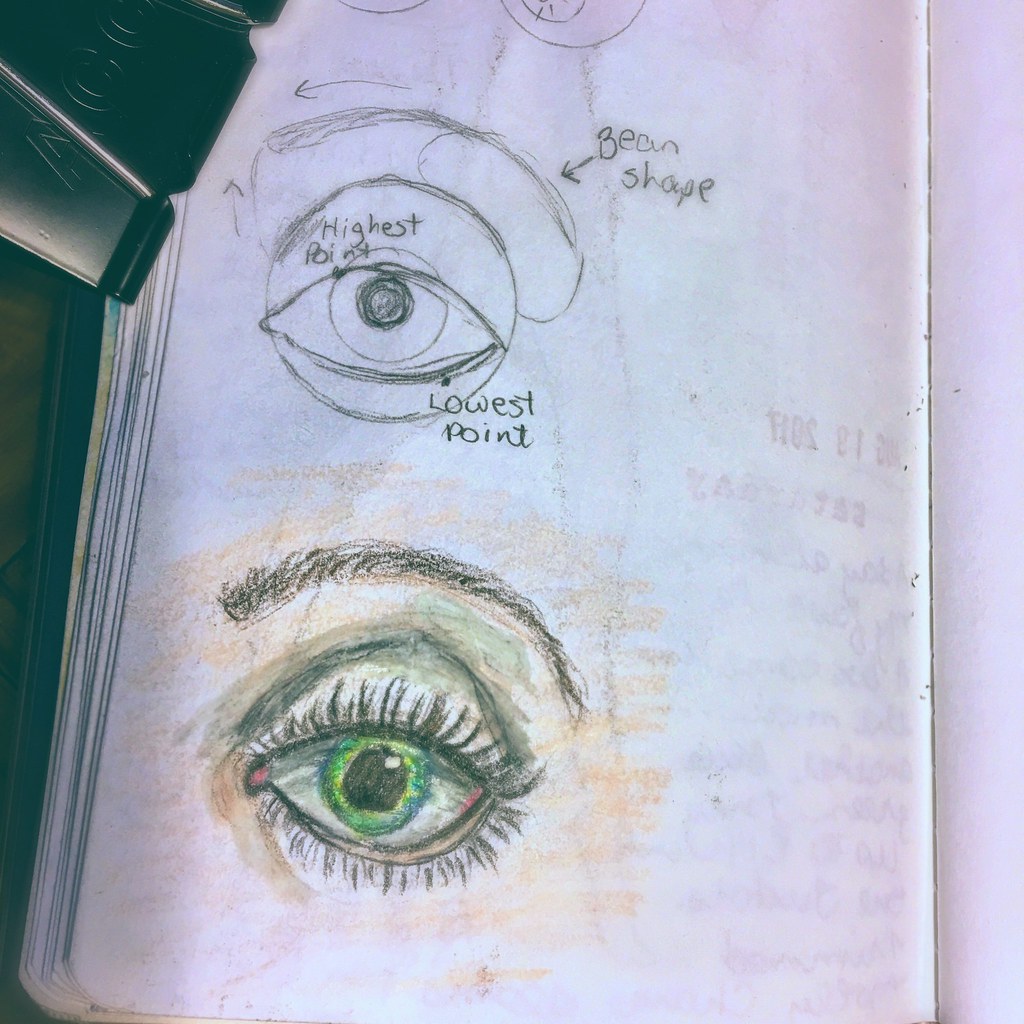In this detailed sketch, we observe a page from a sketch pad adorned with multiple drawings of eyes. The top portion of the page features a schematic illustration of an eye, characterized by its overly round shape and annotated with instructional notes. These annotations provide guidance on eye structure, including labels such as "bean shape that's pointed at the eyebrow," "highest point," and "lowest point."

Below this instructional sketch, there is a meticulously detailed drawing of a realistic eye, presumably created by following the guidelines above. This eye is richly colored, showcasing a vibrant green iris complemented by delicately drawn eyelashes and a well-defined eyebrow. The contrast between the schematic and the realistic eye highlights the instructional purpose of the initial drawing, serving as a precise guide for achieving the more lifelike rendition.